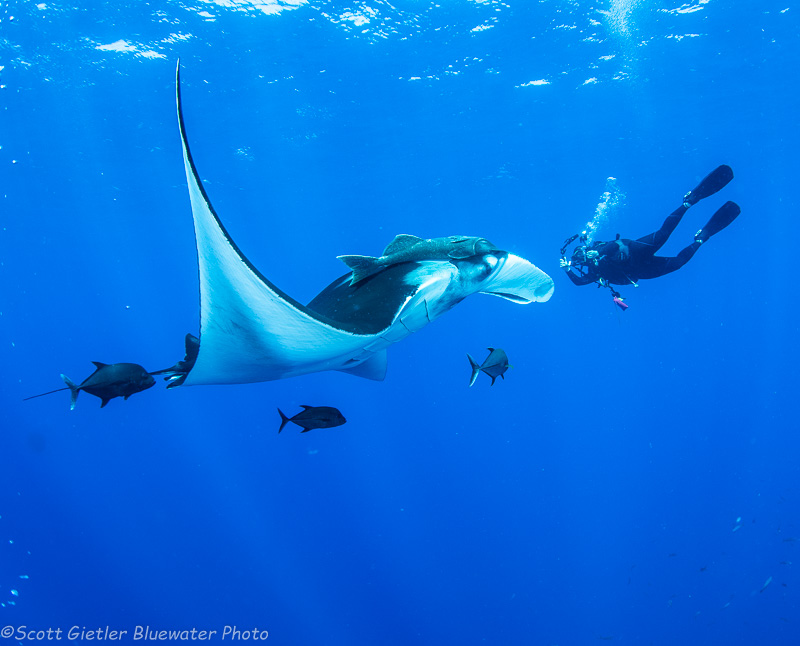The underwater photograph, taken by Scott Gietler of Blue Water Photo, captures an elaborate marine scene bathed in a rich blue hue. Light rays penetrate the water, casting patches of illumination that hint at the surface above. The central focus is a large stingray, gliding effortlessly with one fin pointed toward the surface and the other extending horizontally. Its topside is a dark hue in sharp contrast to its stark white underside. Atop the stingray rides a remora, latched securely for the journey.

Beneath and around the stingray, various fish swim, including three positioned directly below it, and one closer to the forefront near the diver. These fish are mostly dark-colored with white edges on their tail fins, characterized by their V-shaped tails and rounded backs.

On the right side of the frame is a scuba diver in a black wetsuit, complete with fins and a face mask from which bubbles rise, suggesting recent exhalation. The diver's hand is positioned in front of their face, possibly indicating they are taking a photograph. This serene and mesmerizing underwater tableau showcases the stingray's graceful swim, accompanied by a host of marine life and the observant diver, creating a dynamic and intricate marine snapshot.